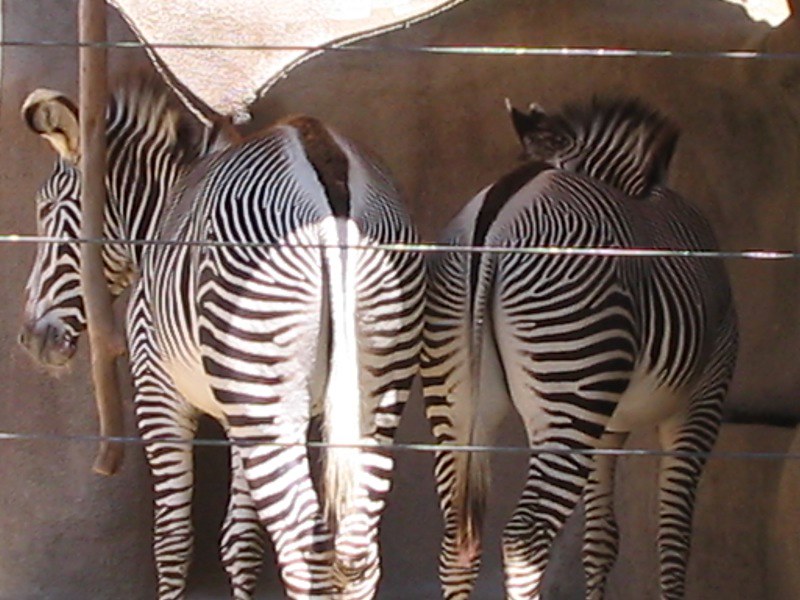This sepia-toned photograph, likely taken outdoors possibly at a zoo, features two zebras standing side by side with their backs to the viewer. The zebra on the left is slightly more illuminated by sunlight, creating an oval highlight patch on its back and casting its tail in bright light, making the tail's details indistinct. This zebra's head is turned to the left, profile just visible along the edge of the image, revealing its dark muzzle and eye. The zebra on the right is more shaded, with its head tucked in and barely visible except for its erect mane. Both zebras display the striking characteristic black and white stripes, with white underbellies and slender tails featuring a central black stripe. Additionally, their strong hind legs are prominent, standing cut off at the knees. The setting seems enclosed with three strips of thin metal wire fencing running horizontally across the image, possibly confining them within the area. The backdrop suggests a den-like structure or a shaded enclosure, while a cloth piece and a wooden or metallic pole hang from the top left part of the image, adding to the sense of a controlled habitat.